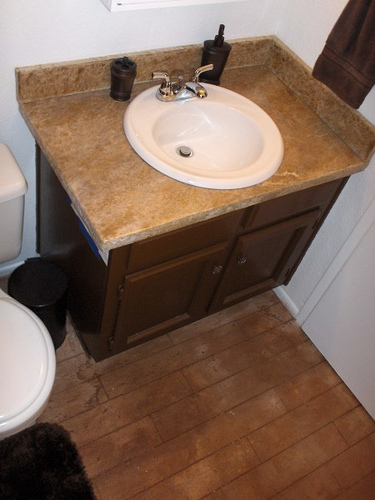This photograph captures a bathroom scene from the perspective of a person standing slightly to the left, near the front of a white toilet. The sink, positioned against the wall on the right, features a standard white basin with a silver faucet fixture that includes built-in handles, designed as a single, cohesive unit rather than separate pieces. 

A dark brown soap dispenser and a matching toothbrush holder rest on the gray-brown granite countertop, adding a touch of contrast to the bathroom's color scheme. The faded, wooden floor beneath shows signs of wear, with white water stains interrupting its otherwise brown hue. 

In the foreground, a bath mat lies on the floor in front of the toilet, suggesting that the photographer was standing on it, looking slightly down and to the right. A black wastebasket with a matching lid sits between the toilet and the sink, maintaining the room's neat appearance. 

The base of the sink comprises dark wooden cabinets adorned with metal doorknobs, adding a solid and functional element to the overall design of the bathroom.